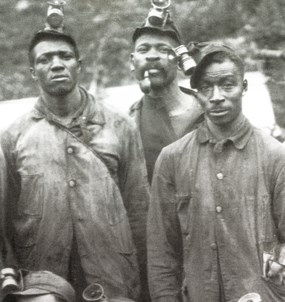A black and white outdoor photograph depicts three African American miners, their serious expressions captured under natural light. The primary focus is on these men, two standing in the front and one slightly behind them. They wear miner's helmets equipped with lights, hinting at the dark environments they work in. The miner at the center sports a thick, full mustache and holds a pipe in his mouth, adding a personal touch to his rugged appearance. All three are dressed in heavy, long-sleeved clothing, suggesting a cold day, while the glints of sunlight accentuate their weariness. In the lower left corner, the top of another man's head with a hat is partially visible. Their surroundings are ambiguous, possibly featuring a white backdrop with trees or a scene sprinkled with snow. The men's darker brown skin and the dust on their clothing underscore their labor-intensive occupations, painting a vivid picture of their challenging lives.